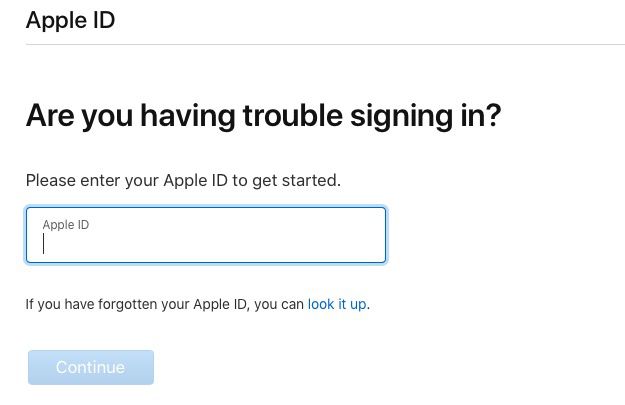The image displays a webpage graphic for Apple's sign-in assistance. In the top left corner, the text "Apple ID" is prominently featured in thick, black font with both letters capitalized and spaced closely together as a single unit. Beneath this, there is a thin horizontal line. Below the line, in a larger font, the text "Are you having trouble signing in?" is presented, with an emphasized, capitalized "A". Further down, there is an instruction line that reads, "Please enter your Apple ID to get started."

A text input field, outlined in blue, is provided for users to enter their Apple ID. Above this field, there is a reiteration of "Apple ID" followed by a separator line. A note below indicates, "If you have forgotten your Apple ID, you can look it up," with "look it up" formatted as a clickable blue hyperlink.

Near the bottom, there is a button with a blue background and the word "Continue" in white text. The "C" in "Continue" is capitalized. This button is currently inactive and will become functional once the Apple ID is entered. The entire page maintains a clean, minimalist aesthetic with a white background.